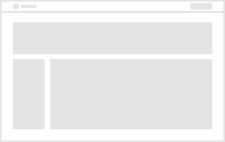This small image appears to be an icon representing a generic webpage layout, intended as a placeholder or a schematic. On a white background, several light gray boxes are arranged to suggest different elements of a typical website. 

In the top left corner, a small gray circle sits alongside a horizontal gray bar, likely representing a website logo or favicon and a search bar. The top right corner features a slightly larger horizontal gray bar, which might symbolize navigation links like "login" or "shopping cart."

Just below this header section is a long horizontal gray bar, indicative of a main menu or navigation bar for the website. Centrally located on the image are three prominent light gray boxes: one large horizontal box at the center top possibly for a main title or feature section, and two slightly smaller boxes stacked beneath it.

In the bottom left corner, a small vertical gray box might represent a sidebar category or additional links, next to a larger horizontal gray box on its right which could stand for content preview or promotional space.

All of these gray boxes are separated by white lines, emphasizing their distinction from one another. This image, devoid of any actual text, graphics, or photos, serves as an illustrative symbol of a basic webpage structure.